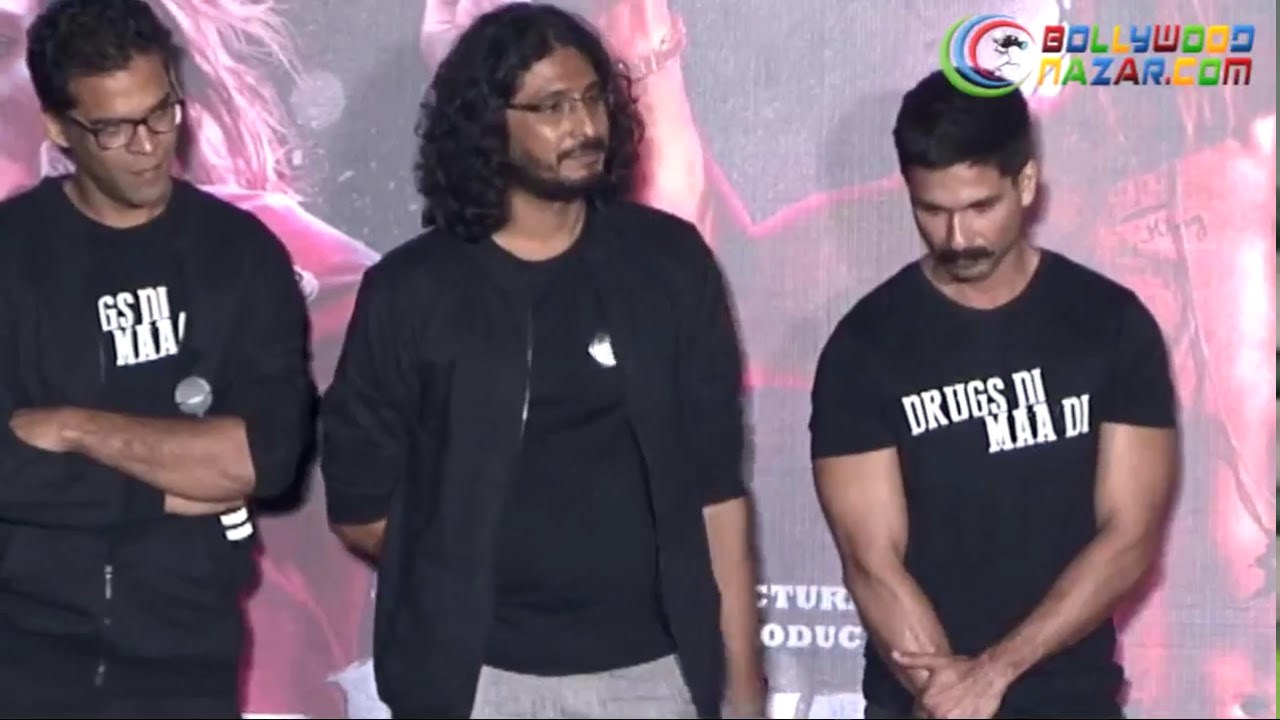This image features three young Indian men standing in front of a partially visible poster, likely connected to Bollywood, as indicated by the multicolored "BollywoodPlaza.com" logo in the upper right-hand corner. All three men are dressed in black attire, focusing on their shared theme and expressions.

Starting from the left, the first man has his arms crossed over his chest, holding a portable microphone in his right hand under his left arm. He is wearing a black hoodie over a black t-shirt with partially visible white text ("drugs," "me," and some additional letters). He has dark hair and glasses and is looking off to his left (our right).

The man in the center has shoulder-length, wavy hair, glasses, and a short beard. He sports a black jacket over a black t-shirt and light-colored pants. He, too, is looking slightly leftwards with a neutral expression.

On the far right, the third man stands with his hands clasped in front of him. He is muscular and has short hair with a mustache. His black t-shirt displays the white text "drugs," "dimadi" or possibly "drugs NI maa di," where the full interpretation remains unclear. He is looking downward, creating a contemplative appearance.

The backdrop features indistinguishable figures and colors, conveying a busy or vibrant scene. The overall ambiance, coupled with the cohesive choice of attire and the Bollywood connection, suggests these men might be figures or participants in the Indian cinema scene.